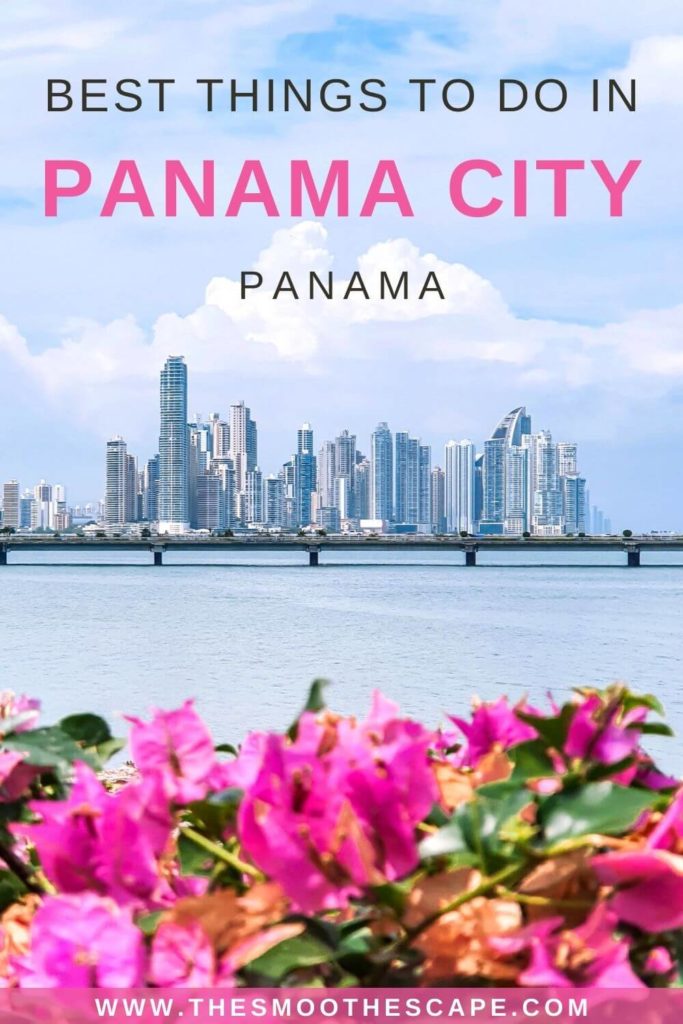The image is a screenshot of a visually striking title splash page for an article titled "Best Things to Do in Panama City, Panama". The presentation resembles a portrait-oriented book cover, emphasizing an engaging and structured aesthetic. Dominating the center of the image is a breathtaking view of Panama City, featuring its sprawling skyline, which subtly suggests the vibrancy and dynamism of the city. Complementing this urban panorama is a prominent long bridge stretching across a serene expanse of water. The bridge sits relatively low over the water, possibly too low to allow the passage of large boats beneath it.

In the foreground, a cluster of vibrant pink flowers adds a touch of natural beauty and color contrast to the otherwise urban-themed image. Some additional flowers, in shades of green and brown, further enrich the scene. At the top of the cover, the title "BEST THINGS TO DO IN PANAMA CITY, PANAMA" is boldly displayed, with "Panama City" highlighted in an eye-catching pink color, emphasizing the destination's appeal. 

The bottom of the image features a pink banner that includes the website address "www.thesmoothescape.com", suggesting the origin of the content and inviting readers to explore further.